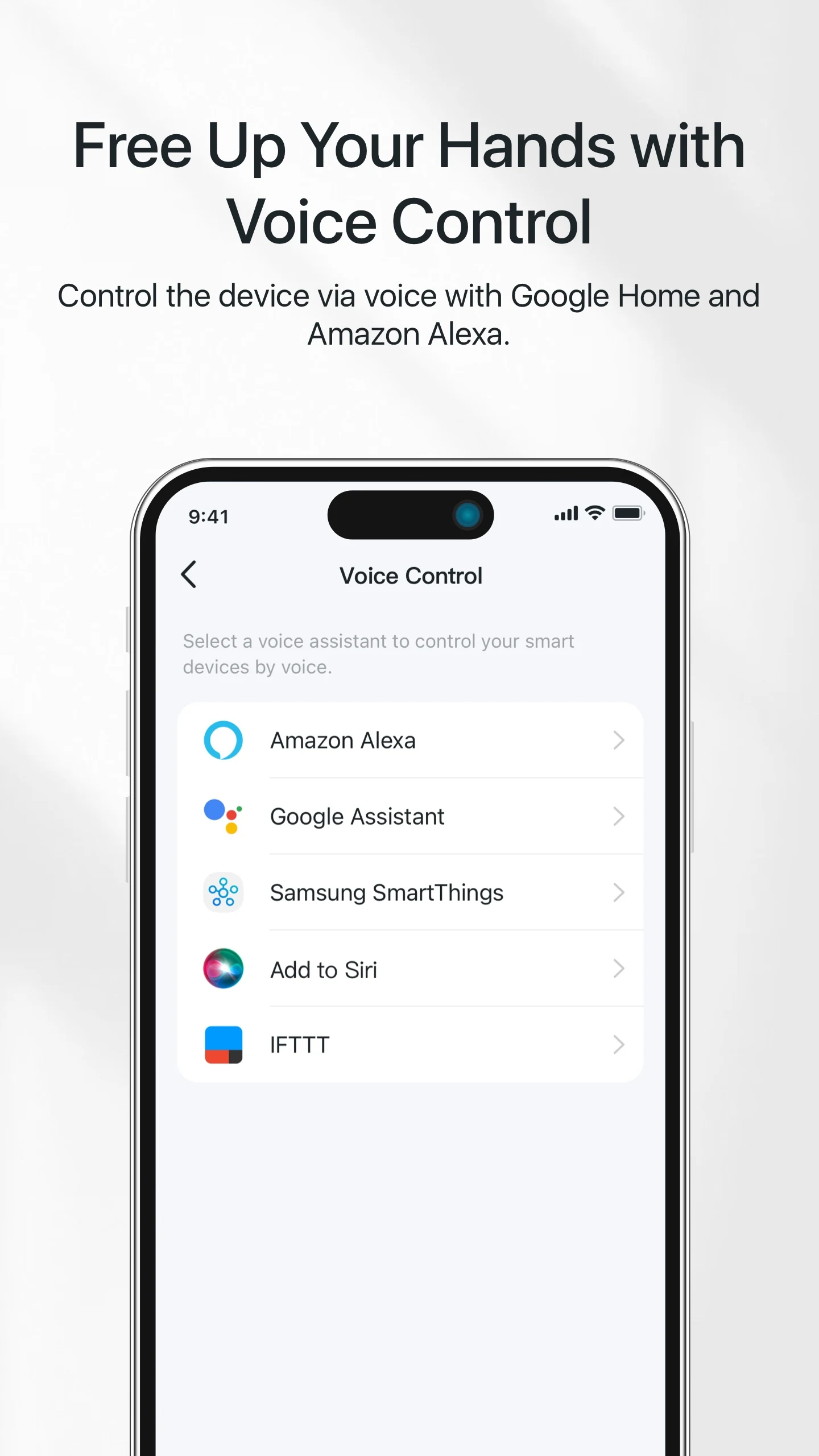The image features a predominantly white background with a subtle gray hue and delicate shadows. Central to the composition is a smartphone, aligned vertically from the bottom to the middle of the frame. At the top of the image, bold black text proclaims, "Free your hands with voice control." Beneath this, smaller, non-bolded black text elaborates, "Control the device via voice with Google Home and Amazon Alexa." The smartphone's screen, which is visible, displays a white interface with the heading "Voice Control" at the top. Below this heading are icons for various voice control apps, including Amazon Alexa, Google Assistant, Samsung SmartThings, Add to Siri, and IFTTT.